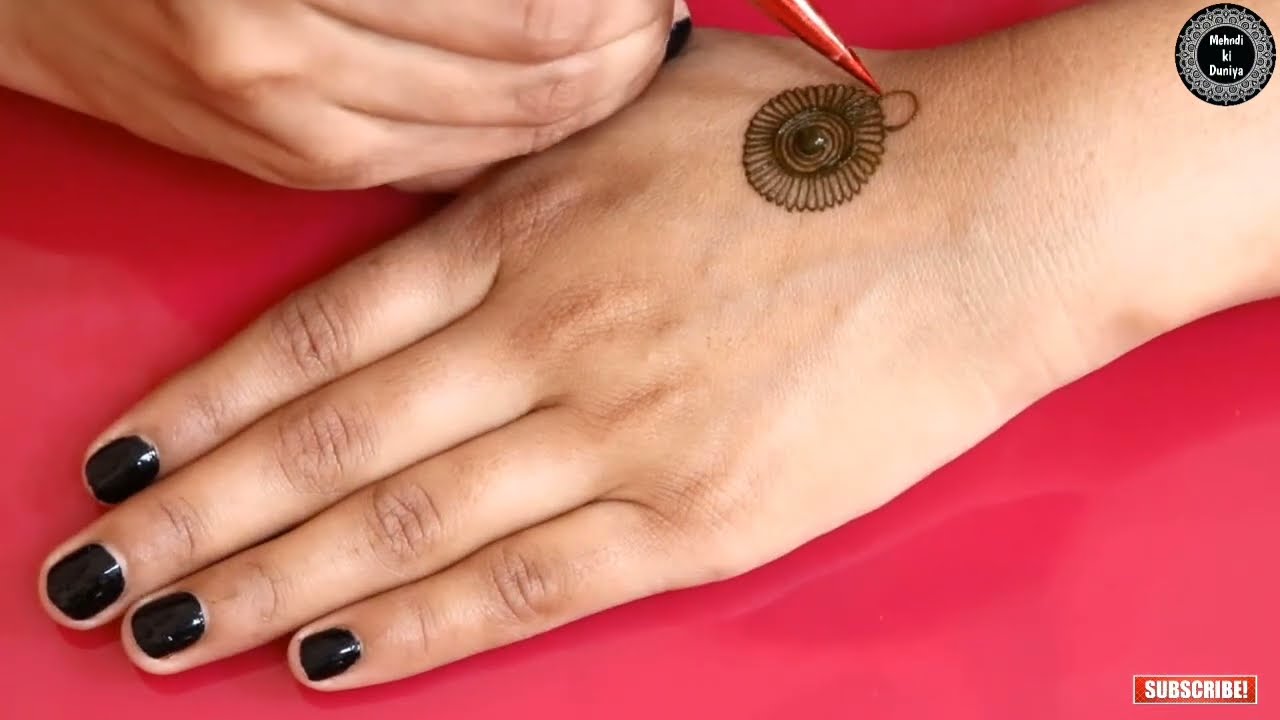The photograph captures a close-up view of a slightly tanned left hand, adorned with shiny black nail polish, lying flat against a bright, shiny red background. This hand extends from the top right corner of the image down to the bottom left, where its fingertips rest. A precise henna design, featuring a spiral surrounded by delicate, thin petals and beginning a new petal layer, is being illustrated on the back of this hand, just above the thumb area. This intricate henna work is being applied by another hand, which is partially visible with knuckles and the back of the hand shown, leaning against the first hand. The tools used for the henna appear reddish and are seen poking out from the top of the image. In the bottom right corner, the word "subscribe" is prominently displayed, while the top right corner features a pixelated text reading "MEHEDI K-L DUNIYA."